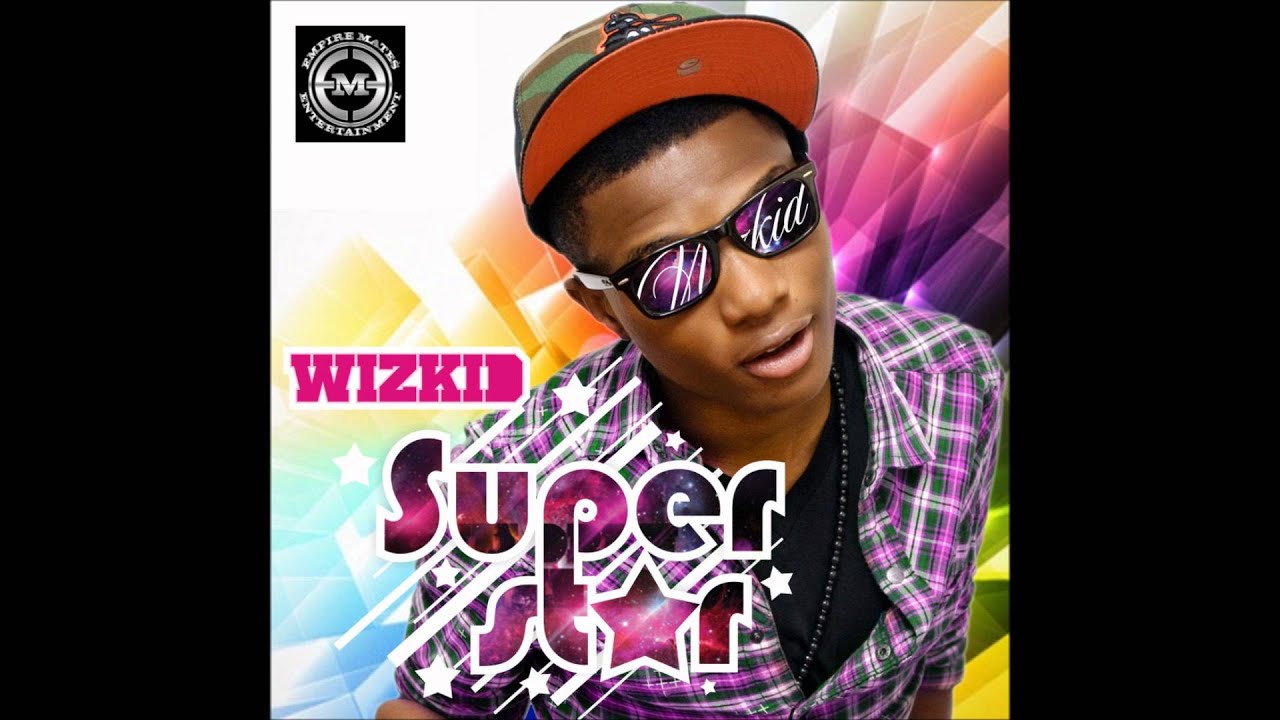The image is a vibrant advertisement featuring a young African-American teenage boy, positioned centrally within a square frame, bordered on both sides by black strips. He is dressed in a purple plaid shirt layered over a black t-shirt, wearing a green cap with a red bill and an indeterminate logo. A thin silver necklace hangs down over his chest. The boy sports dark reflective sunglasses, with "wiz kid" displayed on each lens. Across the image, "Whiz Kid" appears in smaller purple uppercase font, and below it, "Superstar" is prominently displayed in larger purple uppercase and lowercase letters with white borders, featuring a star symbol in place of the "A". The background is adorned with prismatic colors, adding a dynamic feel.

In the upper left corner, there is a circular logo that reads "Empire Mates Entertainment" in a black and white compass-style motif. This design contributes to the overall aesthetic, which blends modern and retro 60s typography with star lights and stage light effects enhancing the "Superstar" text. The image conveys a vibrant and dynamic energy, possibly promoting a music artist or a video game.